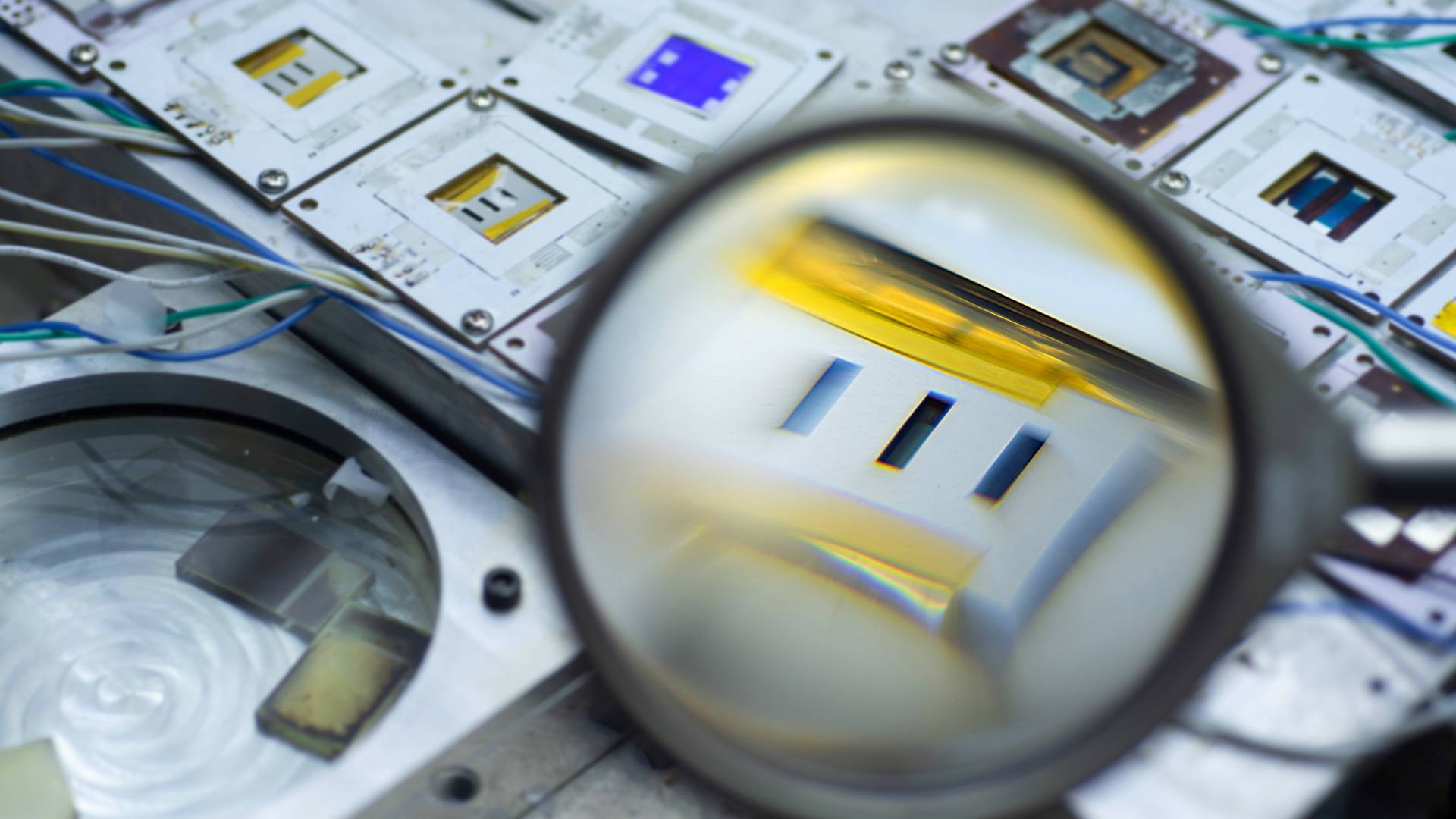The image showcases a detailed close-up of an electronic device, highlighted by a magnifying glass positioned on the right side. The magnifying glass magnifies a specific section of a microchip, revealing three parallel elongated rectangular slots on a white board, some of which are secured with yellow tape. The backdrop reveals an array of similar microchips, each varying in design—some featuring vibrant centers in blue and purple, others with yellow or blue backgrounds. Additionally, there are various plates with four corners, each mounted with metal screws. At the bottom of the image, a different electronic device is visible, connected by a combination of blue, white, and green wiring. This wiring appears to link the device to the microchips beneath the boards, providing a complex network of electronic components. The overall scene is a meticulous exploration of intricate computer hardware, emphasizing the fine details and interconnections within the composition.